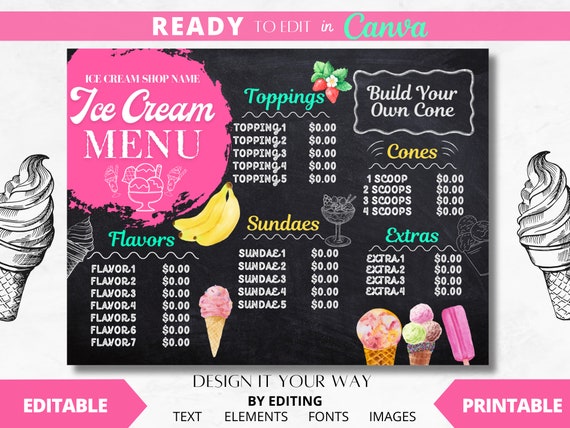The image features an editable and printable ice cream menu template from Canva. Dominated by a central blackboard design, the menu is highlighted with pink accents. At the top of the image, a pink bar states "Ready to edit in Canva," complemented by arrows at the bottom corners indicating "editable" on the left and "printable" on the right. The blackboard menu layout includes placeholders for various ice cream elements: flavors, toppings, cones, sundaes, and extras. Flavors have a photorealistic banana illustration, while the toppings section features red strawberries with a blossom and leaves illustration. Scattered around are images of ice cream cones and popsicles, adding a realistic touch. "Ice Cream Menu" is prominently displayed on a pink splash on the left side. Framing the menu are simple black and white drawings of soft serve ice cream cones on either side. The overall design invites customization with text, elements, fonts, and images to suit any ice cream shop's needs.